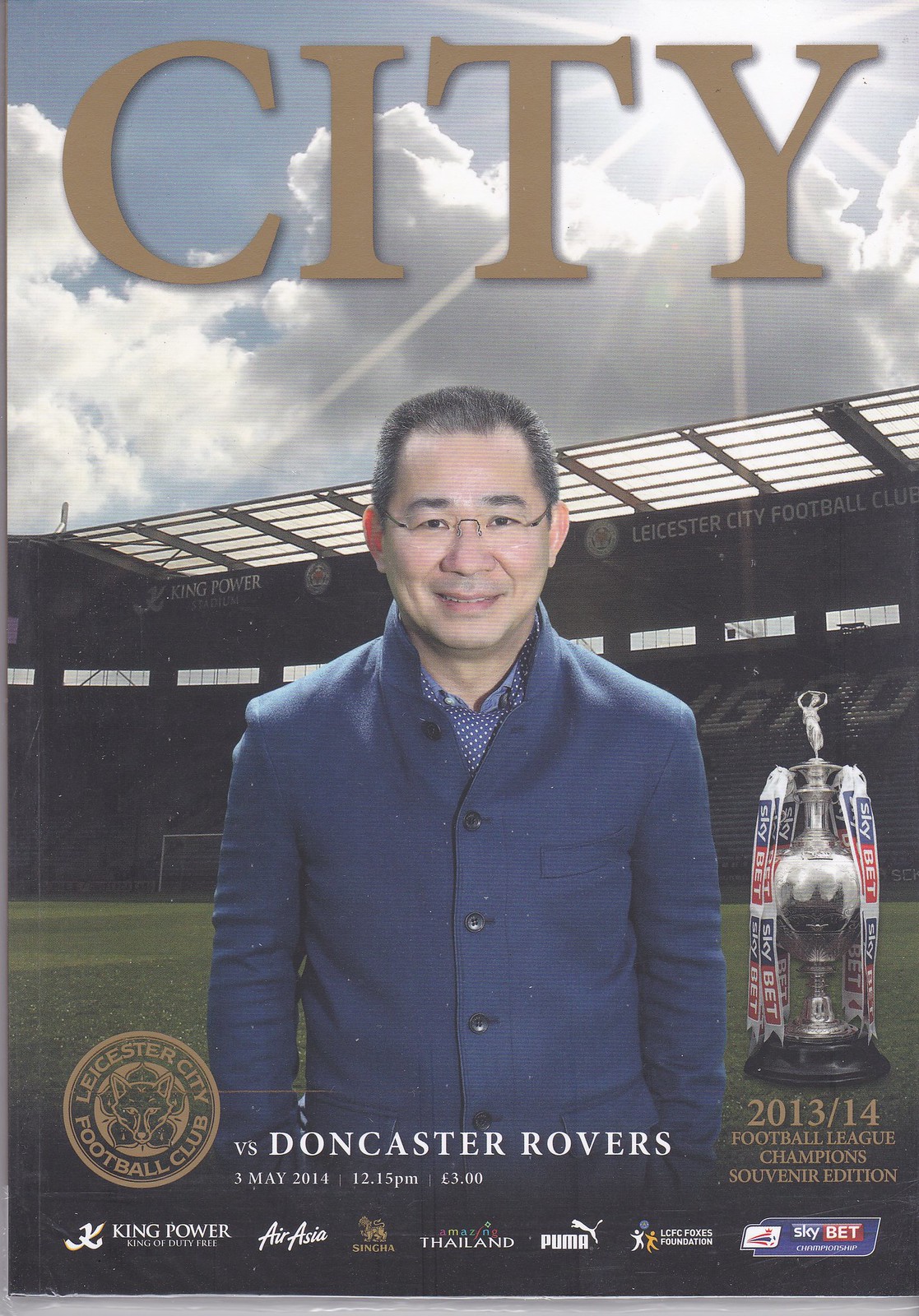The cover of this sports magazine features the title "CITY" at the top in large capital letters, set against a background of clouds with sun rays piercing through. Dominating the center is an older Asian man with short black hair, wearing glasses, and dressed in a blue button-up coat over a shirt and tie. Behind him, the Leicester City Football Club Stadium can be seen with its stadium seats, lights, and roof partially visible. To the man's right is an image of a trophy with the text "2013/14 Football League Champions Souvenir Edition" beneath it. Across the man's stomach level, the text "Doncaster Rovers" is prominently displayed in white, accompanied by a golden emblem to the left. Further details include the date "3rd May 2014, 12:15 PM" and the price "three pounds." At the very bottom, there are around six advertisements featuring logos such as Puma, King Power, and Skybet, although some are difficult to read. In the bottom right-hand corner, there is a small box with a blue background and some unreadable text.